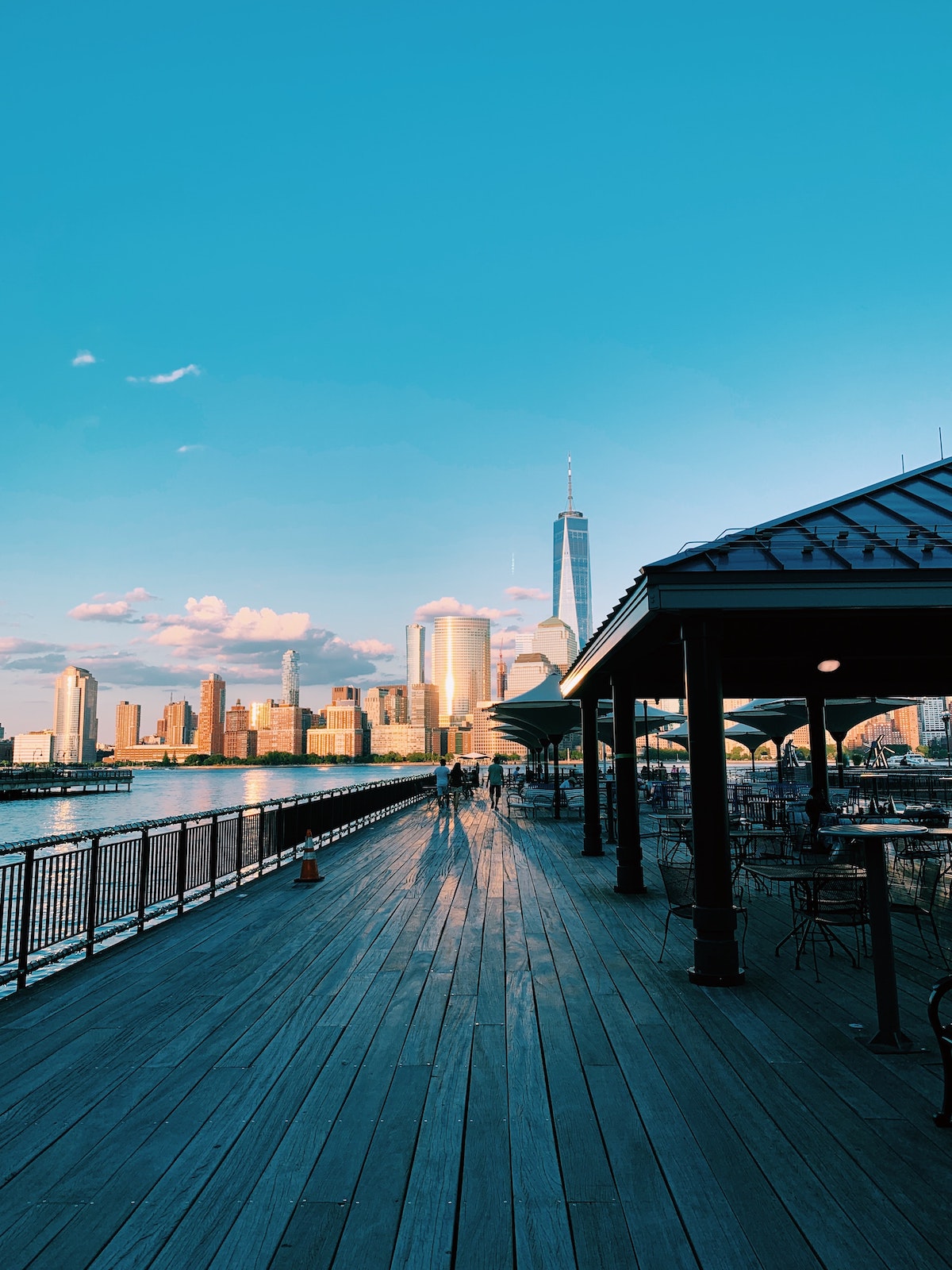This detailed picture captures a scenic view of New York City, prominently featuring the Freedom Tower against a clear blue sky with patches of white clouds, bathed in late afternoon sunlight. In the foreground, there's a large pier with a waterside gazebo furnished with tables and chairs. The scene is animated by people walking on the wooden planks of the pier, which is secured by railings, and some are seated under the gazebo, enjoying what appears to be a restaurant setup. The vibrant blue water of the adjoining water body enhances the picturesque seascape, making it a very inviting and lively location.